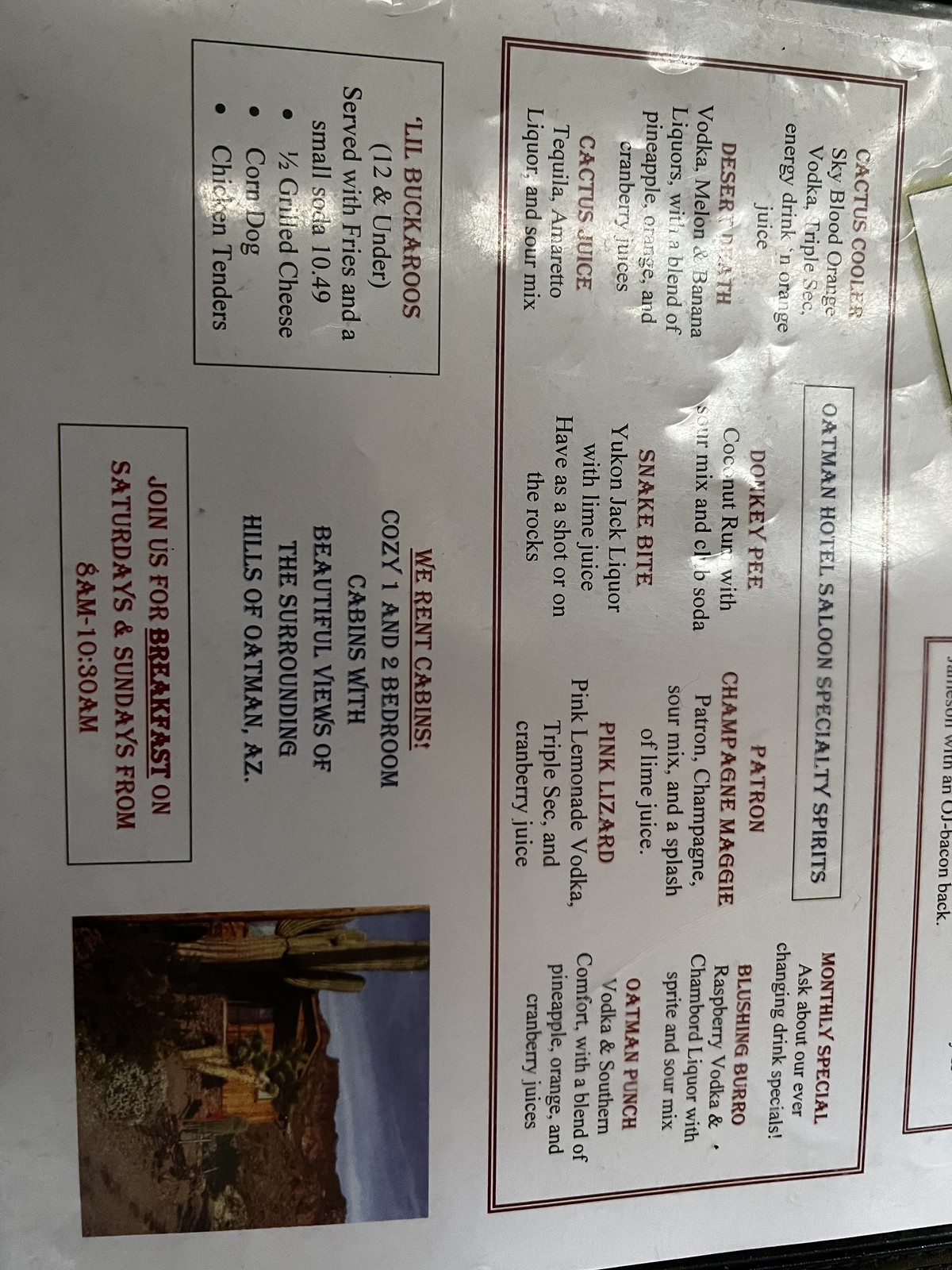The image depicts a glossy, laminated menu turned 90 degrees to the left, making the text appear sideways. The reflective surface of the lamination catches the light, creating a shiny effect across the menu. The menu features a vibrant red text box highlighting a section titled "Oatman Hotel Saloon Specialty Spirits," showcasing an array of mixed drinks such as Cactus Cooler, Desert Death, Cactus Juice, Donkey Pee, Snake Bite, Patron Champagne, Maggie, and Pink Lizard. It also mentions a Monthly Special with options like Blushing Burrow and Oatman Punch.

On the bottom left corner of the menu, which translates to the bottom left of the photo due to its orientation, there's a section labeled "Lil Buckaroos," indicating the kids' menu for children 12 and under. This section details the choices available, including half grilled cheese, corn dog, or chicken tenders, all served with fries and a small soda for $10.49.

Adjacent to the kids' menu is a notice about cabin rentals, advertising cozy one and two-bedroom cabins with picturesque views of the surrounding hills of Oatman, Arizona. The menu also invites guests to join for breakfast on Saturdays and Sundays from 8 a.m. to 10:30 a.m.

In the bottom right corner of the menu, which appears on the bottom left of the rotated photo, there's a color photograph depicting a saguaro cactus against a desert landscape backdrop, with a streaked blue sky and scattered clouds. The exact subject of the photograph is unclear, but it might represent the restaurant or its surroundings.